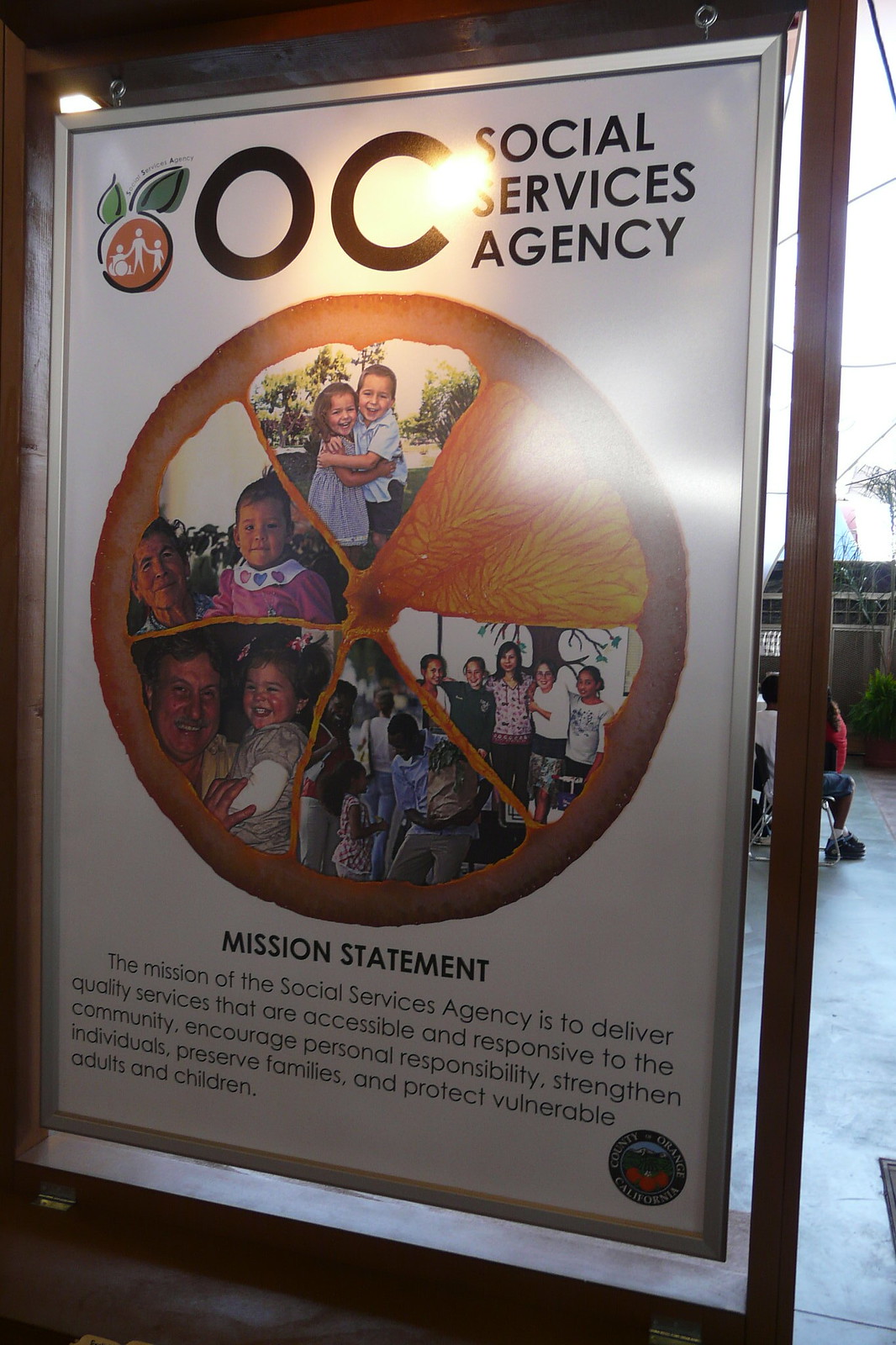The image depicts a large outdoor poster hanging in a brown frame, which serves as signage for the OC Social Services Agency. At the top of the poster, the letters "OC" are displayed prominently. To the right, the words "Social Services Agency" are stacked vertically, each word on a separate line. To the left of the "O" in "OC," there's an illustration of an orange, complete with two small orange leaves at the top and three simple stick-figure people inside it. Below this, a real cutout of an orange is featured, divided into six segments akin to a pizza pie. Each segment contains different photographs depicting families and children engaged in various activities, such as hugging, attending a classroom, and interacting in what appears to be familial settings. The top right segment shows an orange peel, while the other five segments feature images of people. At the bottom of the poster, the words "Mission Statement" are boldly printed in dark black, with a descriptive paragraph below that outlines the agency's commitment to supporting and aiding the community. The background reveals the poster set against an outdoor backdrop, with asphalt ground, chairs, a person seated, a house, part of the sky, and some trees visible, enhancing the community-oriented theme of the poster.